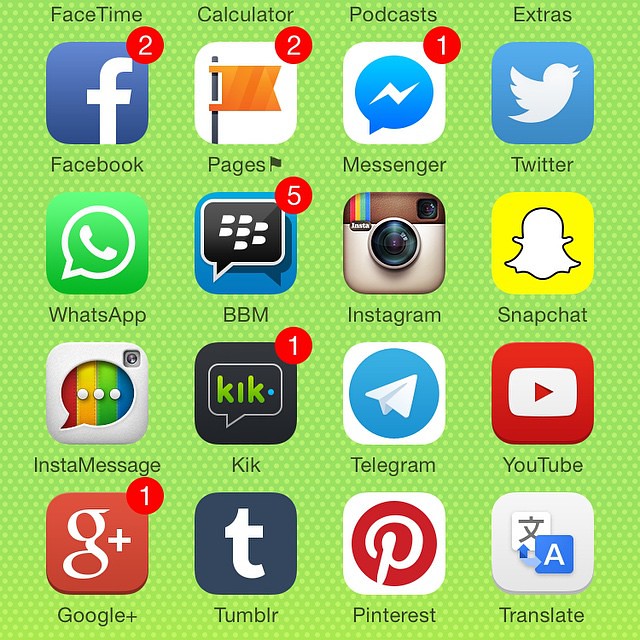Screenshot of a cell phone screen showing a 4x4 grid of app icons against a lime green polka-dotted background. The background features very tiny lighter lime green dots on a darker lime green surface.

**Top Row (Left to Right):**
1. **Facebook** - Two notifications 
2. **Pages** - Two notifications
3. **Messenger** - One notification
4. **Twitter** - Zero notifications

**Second Row (Left to Right):**
1. **WhatsApp**
2. **BBM** - Five notifications
3. **Instagram**
4. **Snapchat**

**Third Row (Left to Right):**
1. **InstaMessage**
2. **Kik** - One notification
3. **Telegram**
4. **YouTube**

**Bottom Row (Left to Right):**
1. **Google Plus** - One notification
2. **Tumblr**
3. **Pinterest**
4. **Translate**

At the top of the screen, partially visible app labels from another row can be seen: FaceTime, Calculator, Podcasts, and Extras.